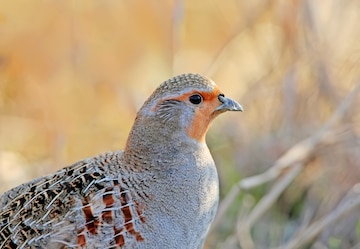This landscape photograph captures a small, detailed image of a bird, possibly a type of quail or partridge, in a natural, woodsy area. The bird's body extends from the bottom left-hand corner to the center of the frame, standing in right profile. Its distinctive features include an orange face with black eyes and a gray beak, while the head is a blend of gray and white. The breast is a speckled gray, transitioning into a heathered gray-brown back adorned with white feather edges and intricate brown and black bars. The background, though blurred, hints at an environment filled with tan, orange, and white hues, suggesting twigs and branches. The bird, fully in focus, stands out clearly against the softly blurred backdrop, highlighting its unique and detailed feather patterns.